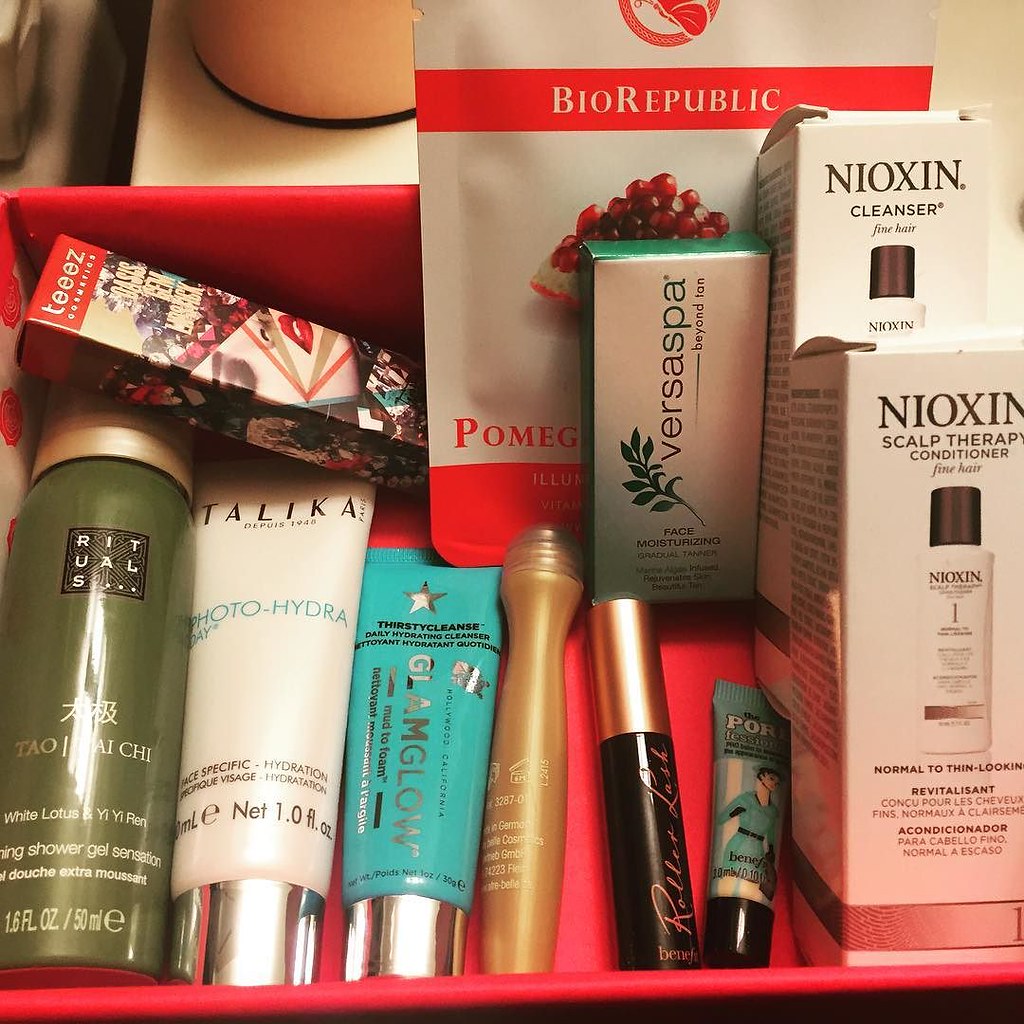In this detailed photograph likely taken in a woman's bathroom, various beauty aid products are meticulously arranged inside a red, square-shaped storage box with a paper-like liner. Positioned on a countertop, the image provides a glimpse into a neatly organized personal care space. 

On the right side of the red box, there are two smaller boxed products from the Nioxin range: one for normal to thin-looking shampoo and the other for conditioner. Moving leftward, a selection of makeup items comes into view, including a mascara and a tube of turquoise pore-covering concealer. The far left section is dedicated to shower products, featuring a shower gel prominently. In the background, a couple of packets can be spotted: one from Biorepublic, which appears to be a pomegranate-themed product, and another indistinguishable boxed item. This photograph offers an intimate look at the variety and organization of beauty products typically used in a bathroom setting.